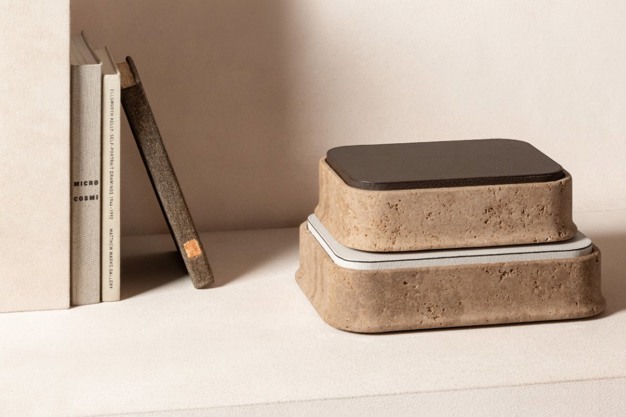In a well-lit room, there's a white wall serving as the backdrop for a scene featuring what looks like the top of a beige or cream-colored bookshelf or table. On the left side, leaning against the far wall, are three monks-like books. The first two books are standing upright: the leftmost book is gray and labeled "Micro, Cosma," while the middle book is white with partially legible text that includes "Math New, Mathellus, Gallery." The third book, brown with a small orange square on the bottom, is angled and resting against the other two. To the right of these books are two brown, cork-colored blocks that resemble platforms or possibly large bookends. The larger block on the bottom features a light gray and white surface, while the smaller one on top has a dark brown top.